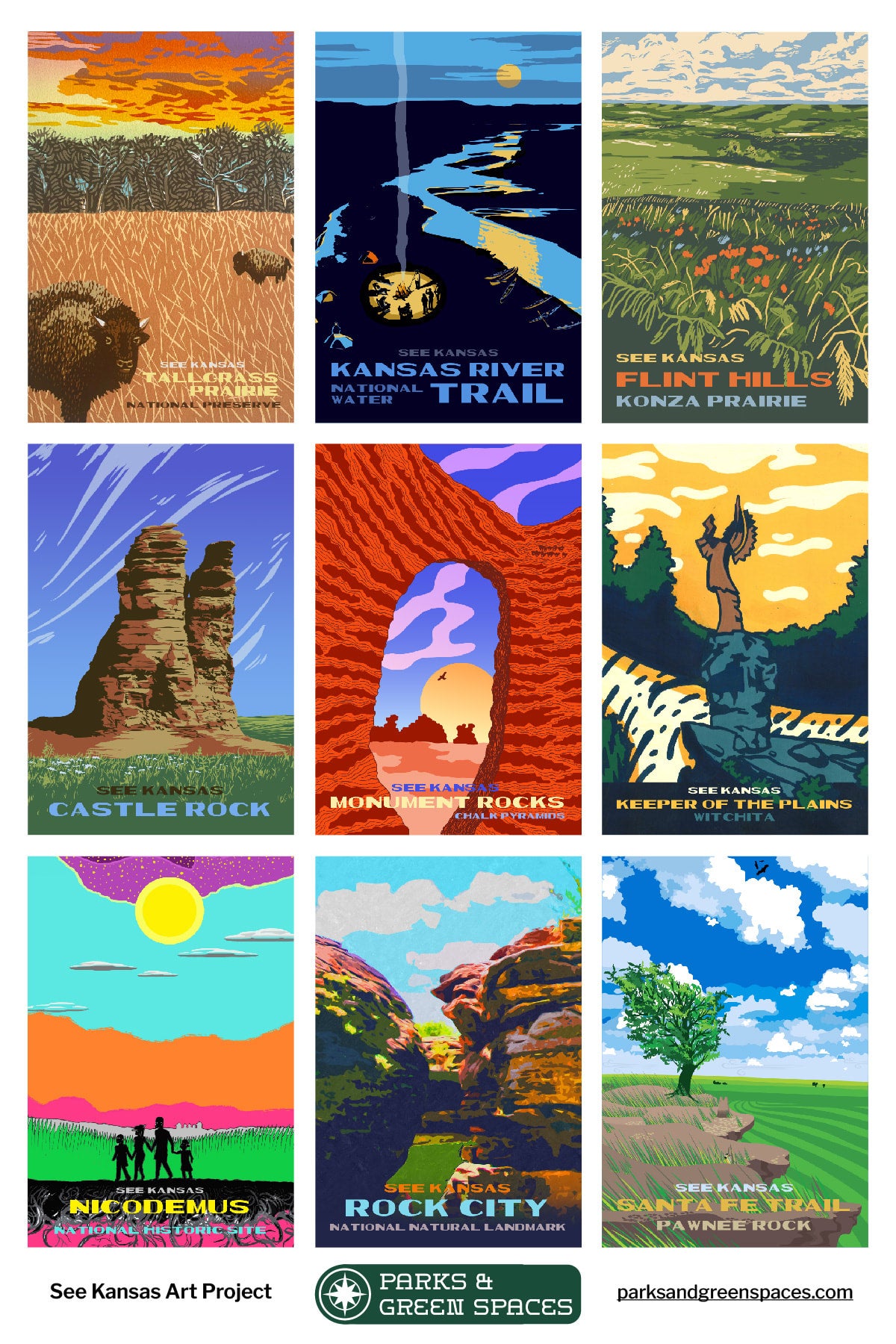The image displays a collection of nine pamphlets arranged in a grid format against a clean white background. There are three rows with three pamphlets in each row. The pamphlets are brightly colored and feature covers with a minimalist, hand-drawn art style, resembling a filtered photograph effect. Each pamphlet focuses on a different scenic or historical location in Kansas, as indicated by their titles. The pamphlet titles include "Kansas River Trail," "Flint Hills," "Santa Fe Trail," "Rock City," among others. Each cover illustration depicts a characteristic scene from the respective locations. For instance, the pamphlet in the top left corner titled "Tallowgrass Prairie" showcases an illustration of a prairie landscape, with two buffalo amidst tall grasses under a sunset sky.